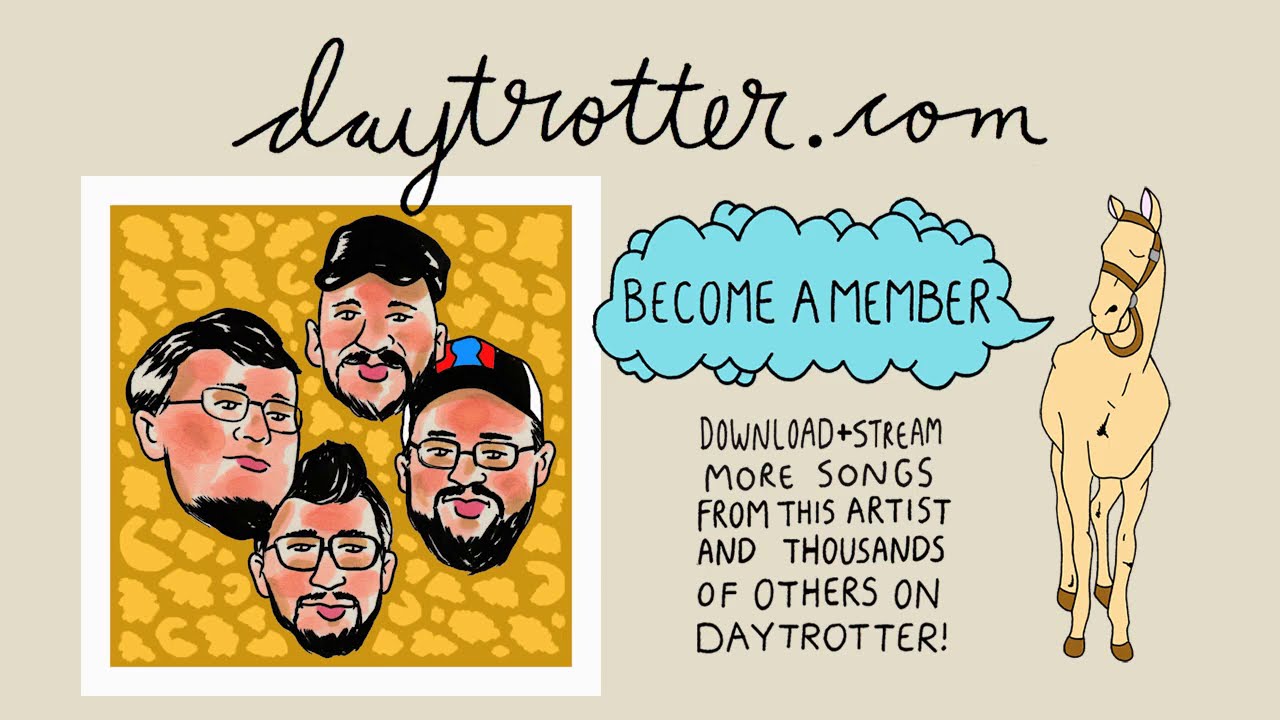The image is a wide horizontal, computer-generated advertisement for daytrotter.com. The background is a light beige, with "daytrotter.com" written in black cursive at the top. On the left side of the image is a white square with a yellow and tan faux cheetah print background. Inside this square are the faces of four men, all with dark hair and facial hair. Three of them wear black-rimmed glasses, and two are wearing dark hats. They have pale to tan skin tones and are likely of European descent. 

On the right side of the image, a tan horse wearing typical horse gear looks towards a blue cloud-shaped word bubble. The bubble contains the text "become a member" in black. Below the bubble, it says, "Download and stream more songs from this artist and thousands of others on daytrotter," also in black text. The overall layout and detailed elements reveal that this is an advertisement for the Daytrotter music platform.